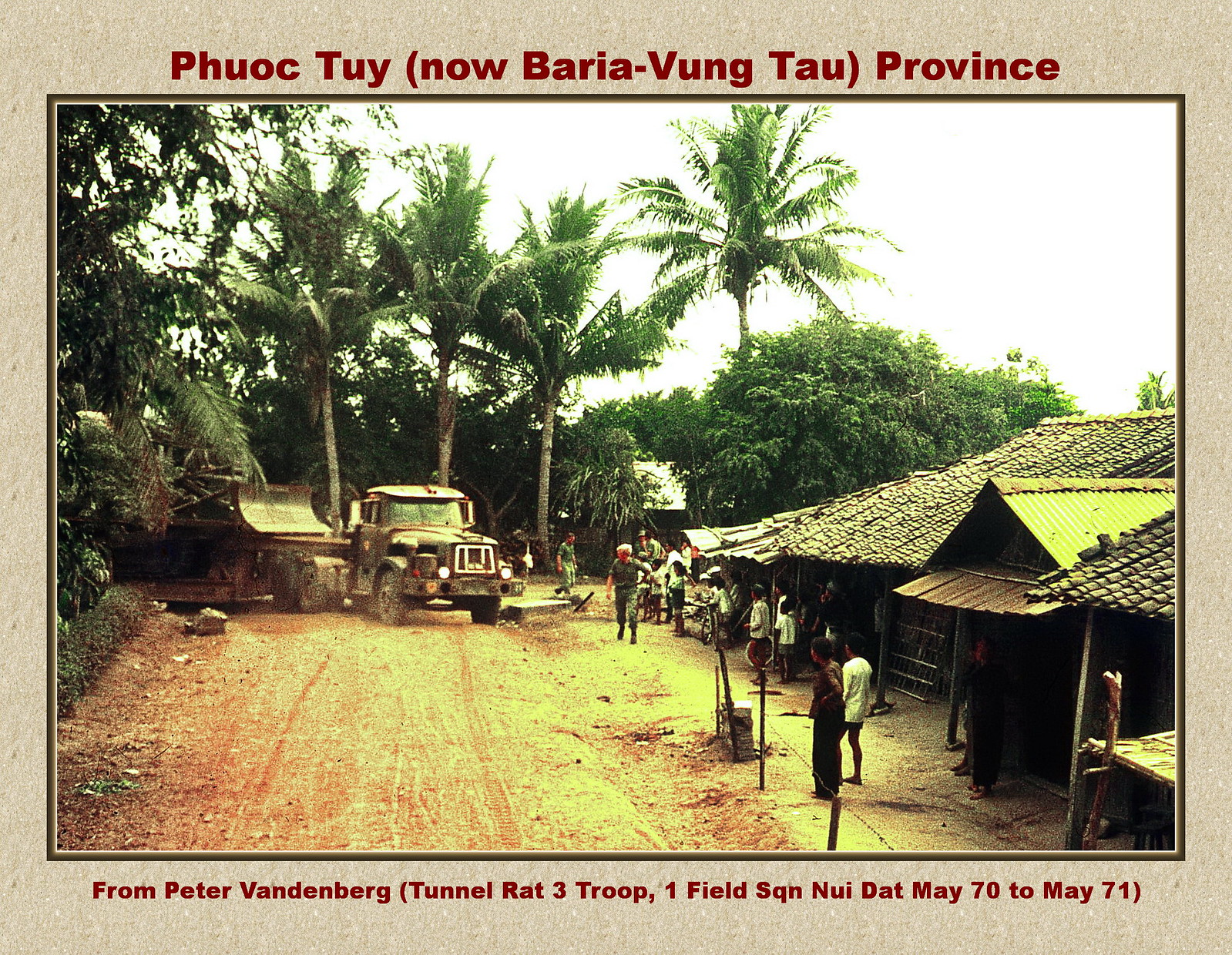The image captures a Vietnam-era photograph, prominently framed by a light sandstone tan border. At the top, in bold red print, is the header "Phuoc Thuy (now Baria Vung Tau province)," with "Phuoc Thuy" spelled as P-H-U-O-C T-U-Y and "Baria Vung Tau" as B-A-R-I-A dash V-U-N-G T-A-U. The bottom text, also in bold red but slightly smaller, reads "from Peter Vandenberg (tunnel rat three troop, one field squadron, Nui Dat, May 70 to May 71)." 

The photograph itself centers on a dirt road. To the right, a row of small wooden houses stands with Vietnamese locals in front, gazing towards the road's end. A towering tropical tree line dots the horizon. Dominating the scene is a large military truck pulling a substantial trailer, with visible military personnel in uniform directing it. Behind the truck sits a Caterpillar Earthmover, resembling a bulldozer. A barbed wire fence separates the huts from the road. The sky, seen in the upper right corner, is a bright, almost blinding white.